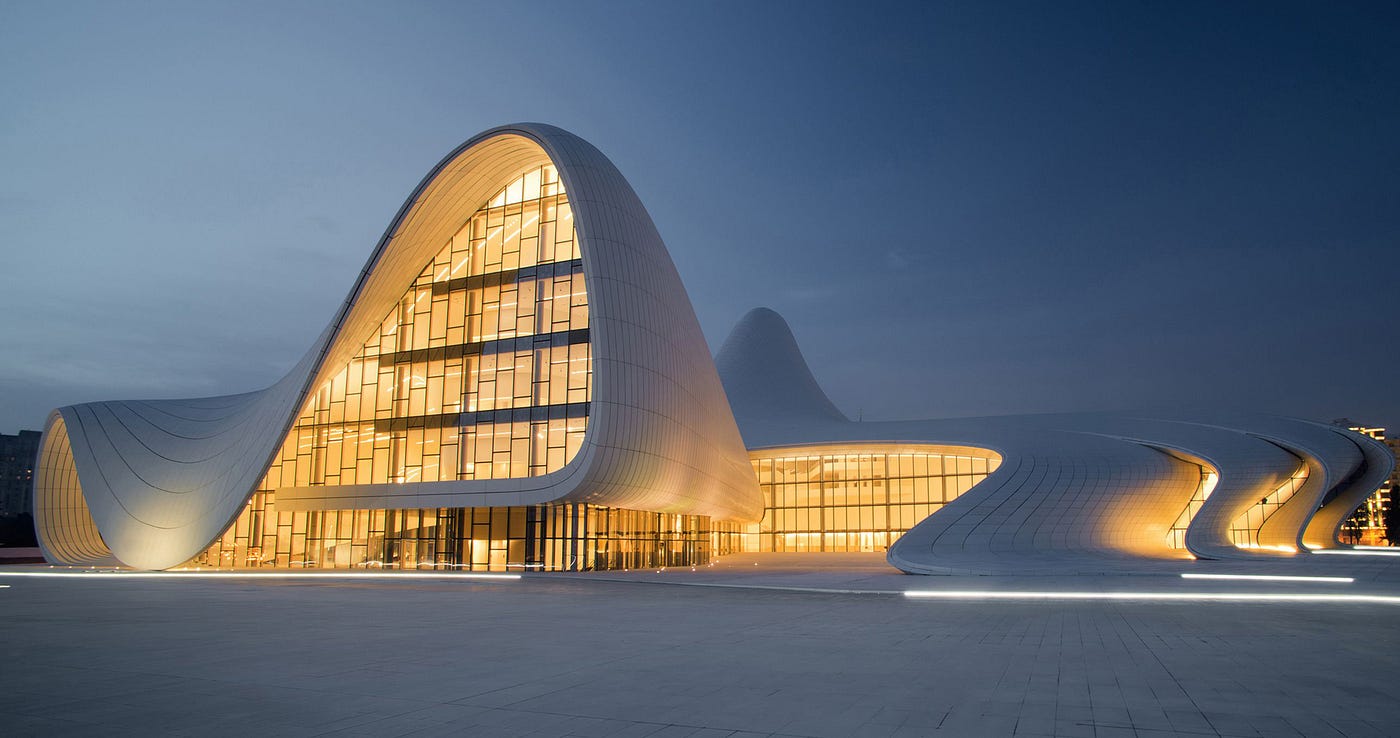This photograph captures the exterior of a uniquely designed building, prominently positioned in the Heydar Aliyev Center, renowned for its modern abstract architecture. The center of the image is dominated by the building's distinctive wave-like design, reminiscent of a crashing wave with its roof arching high before dipping over a series of illuminated yellow windows underneath. On the left side, the building's roof gracefully curves upward and then transitions downward, mimicking the fluid motion of waves. The right side of the image features a series of four ramps, the longest on the left, giving the impression that vehicles could ascend onto the roof. The setting appears to be during nighttime, as the surroundings are dark gray, contrasting with the glowing yellow light emanating from the building's interior through its large, curved windows.